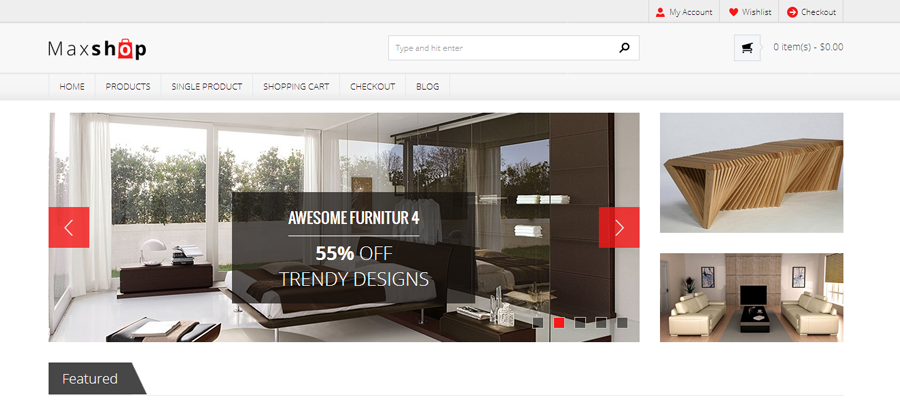**Descriptive Caption for MaxShop Homepage**

The homepage of MaxShop, an online furniture retailer, features a distinctive logo where the "O" in "Shop" is creatively adorned with a red shopping bag. Adjacent to the logo, there is a well-organized navigation bar that includes a search bar and a shopping cart icon indicating zero items. Above this bar, there are quick access options labeled "My Account," "Wishlist," and "Checkout."

Directly below the MaxShop logo, a primary navigation menu offers seamless browsing through buttons labeled "Home," "Products," "Single Product," "Shopping Cart," "Checkout," and "Blog." 

Dominating the header of the homepage is a visually appealing image of a bedroom setup, displaying a complete ensemble including a bed, a dresser, and an armoire. Superimposed on this image is the text "Awesome Furniture 4," followed by "55% off Trendy Designs." This header image is designed for interactivity, equipped with red arrows on either side to allow users to cycle through multiple featured images.

To the right of this main header image are two additional visuals. The first showcases a unique wooden bench constructed from a series of wooden triangles. The second image presents a cozy living room setting, featuring two cream-colored couches facing each other with a sleek black coffee table positioned in the center.